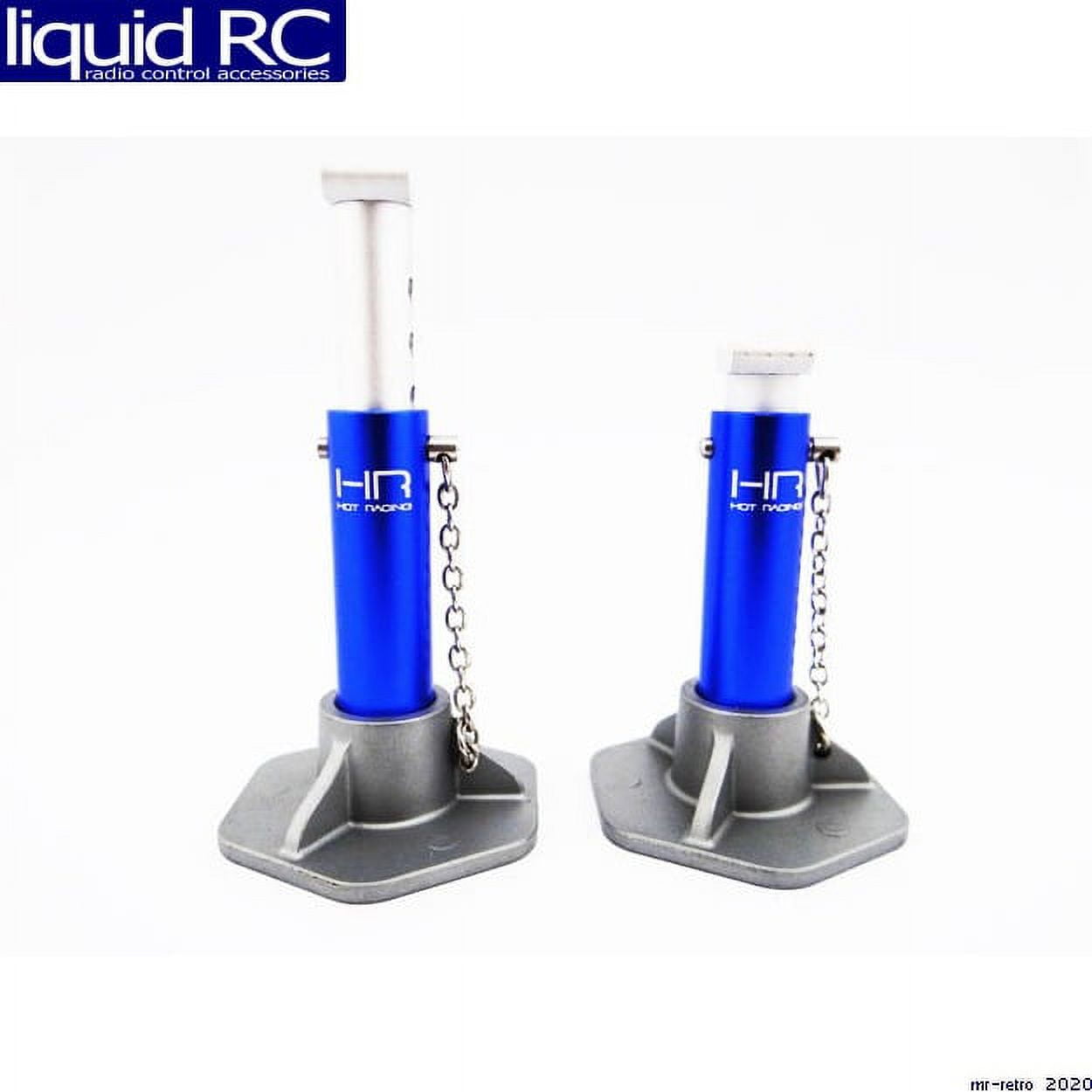The image features a white background with a prominent black and blue rectangular box at the top. Inside this box, the word "liquid" appears in lowercase white letters, followed by "RC" in capital letters. Beneath this, in smaller text, it reads "radio control accessories". The lower part of the image showcases two silver items, each with a hexagonal base and a circular opening above. These openings house tubes that are blue at the bottom and white at the top. The object with the taller tube on the left has the letters "HR", which might stand for "Hot Racing", although the second word is unclear. Both items share the same logo. Additionally, a chain is hanging down from the right side, connecting the blue section with the circular section below. At the very bottom right of the image, "MR retro 2020" is written in black text.